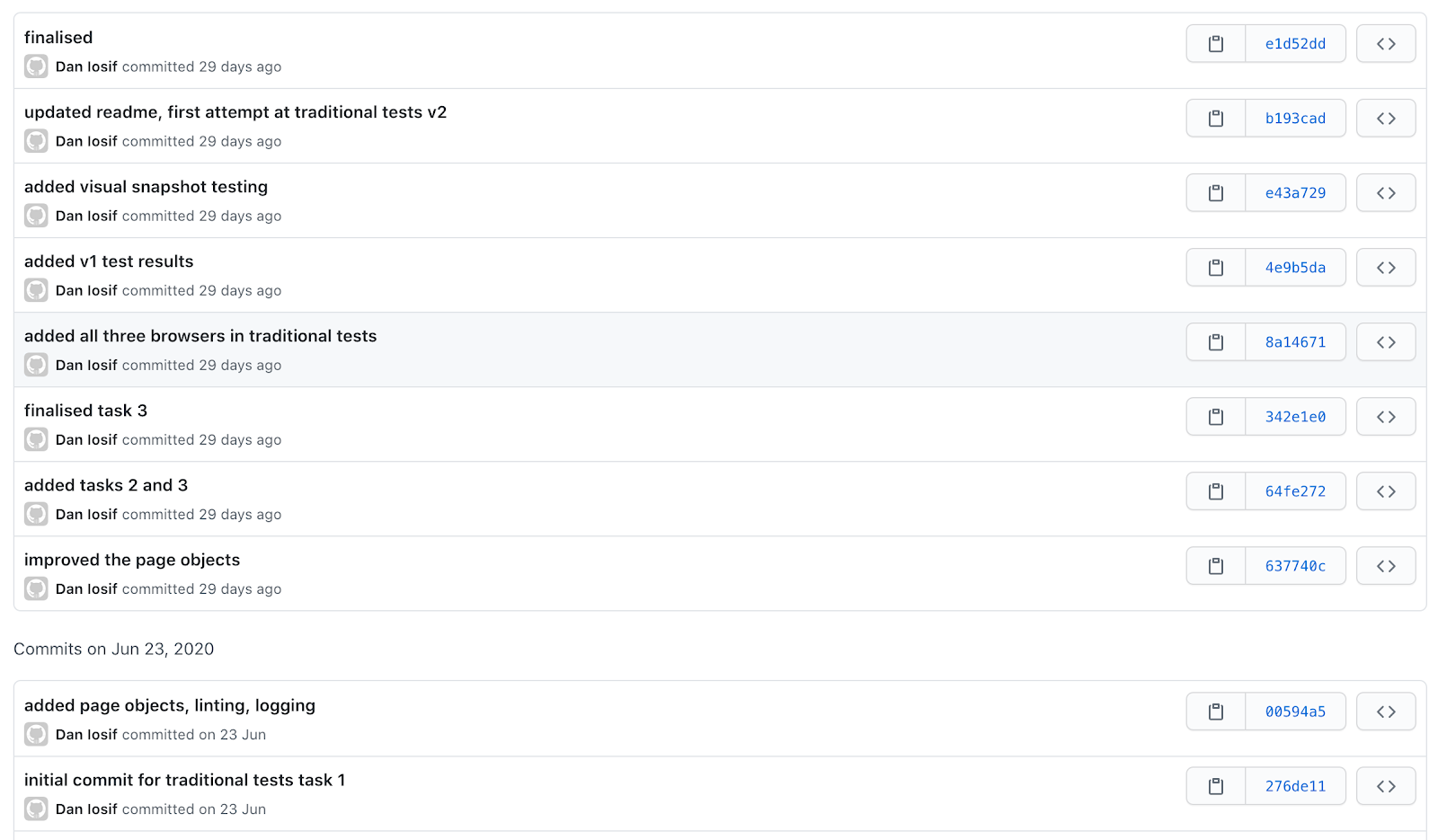The image showcases a minimalist, black-and-white website that lacks a header and a title, making its origin unclear. The site is structured in a straightforward vertical format with sections dedicated to various updates.

Each update is presented in a white box with concise, informative text. The first section is labeled "Finalized, Updated, Read Me, First Attempt at Traditional Test, v2." This section also mentions added visual snapshots and v1 test results, all attributed to Dan Leasiff along with how many days ago each update was made.

Another section is highlighted in gray, detailing more explicit updates such as adding all three browsers in traditional tests, finalizing Task 3, and improving page objects, again credited to Dan Leasiff. Comments from January 23rd, 2020, note the addition of page objects, linting, and logging—also by Dan Leasiff. The initial commit for the traditional test, Task 1, is stated, maintaining the consistent input from Dan Leasiff.

On the right side of the website, there is an image of a box and a set of numbers in blue, flanked by navigation arrows pointing left and right, allowing users to browse through different sections or updates.